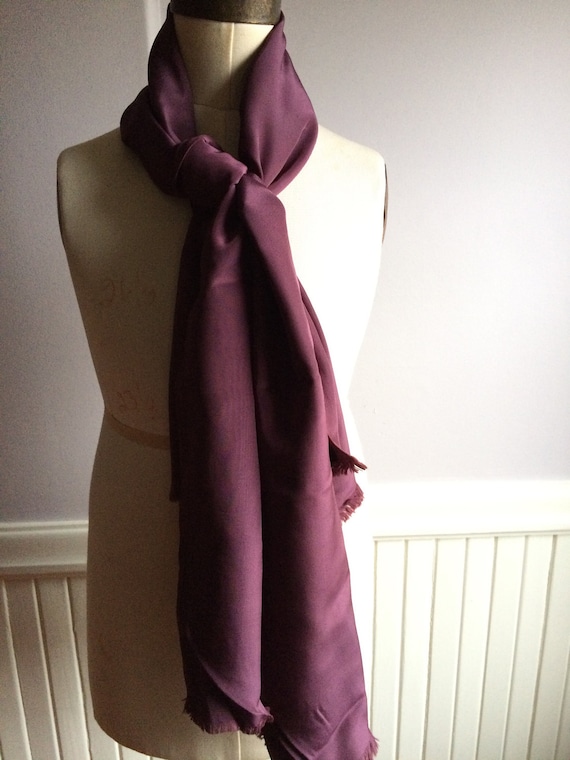The photograph, taken indoors and slightly dimly lit from a window off to the right, captures a dressmaker's mannequin standing against a backdrop of a warm-toned, light gray wall with white beadboard wainscoting that rises approximately a third of the way up. The mannequin, which is a pale beige and lacks both head and arms, features prominently slightly off-center in the left three-quarters of the frame. Draped around the mannequin's neck is a long, flowy burgundy scarf, tied in a simple, loose knot with its frayed edges hanging down nearly to the bottom of the mannequin's torso. The scarf adds a splash of color to the calm, neutral tones of the wainscoted wall and mannequin. The scene is minimalistic, highlighting the elegant simplicity of the displayed scarf.